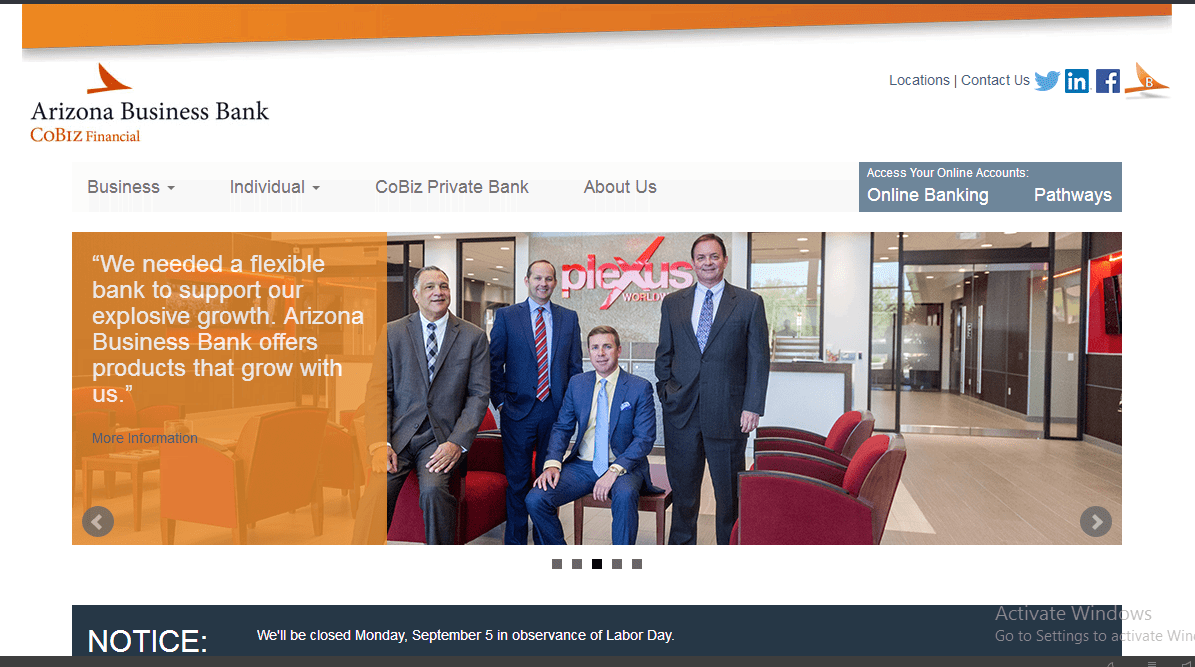**Screenshot of Arizona Business Bank Webpage**

*Description:*

The image is a detailed screenshot of the Arizona Business Bank's webpage, characterized by an orange bezel surrounding the page. 

- **Left Side:**
  - A dark orange wing-like symbol.
  - Below the symbol, the text "Arizona Business Bank" in bold black font.
  - Underneath, "CoBiz Financial" in orange text.

- **Right Side:**
  - "Locations" and "Contact Us" in gray text.

- **Social Media Icons:**
  - A cyan blue bird symbol for Twitter.
  - A dark blue square with an iron symbol.
  - A darker blue square with a white "F" for Facebook.
  - An orange wing-like symbol with a white "B" within.

- **Tabs at the Bottom:**
  - Tabs in black, highlighted by a light gray bezel include:
    - "Business" with a downward arrow.
    - "Individual" with a downward arrow.
    - "CoBiz"
    - "Private Bank"
    - "About Us"

- **Online Banking Section:**
  - On the right, dark gray background with white text:
    - "Access Your Online Accounts" in smaller white font.
    - "Online Banking and Pathways" in bold white text.

- **Image of Individuals:**
  - Next to this section is a photo of individuals with the following descriptions:
    - One individual standing near red chairs.
    - Seated man in a dark gray suit with a white undershirt, dark blue and gray tie, short gray hair with white, light-skinned, looking to the right.
    - A person in a dark blue suit with a red tie with gray and white stripes, light blue undershirt, brown hair.
    - Another person sitting on the edge of a coffee table in a dark blue suit, cream-colored dress shirt, blue tie, brown hair, dark blue dress pants.
    - A final individual wearing a black suit with black pants, dark blue tie, light blue undershirt.

- **Sign Behind Individuals:**
  - Sign in red with the text "PIEXUS WORLOW."
  - Next to the sign, a faded orange rectangle with bold white text, quoting:
    - *"We need a flexible bank to support our explosive growth. Arizona Business Bank offers products that grow with us."*
  - A hyperlink in dark blue font labelled "more information."

- **Notice Section:**
  - Dark blue bezel, bold white text stating "Notice:"
    - *"We will be closed Monday, September 5th in observance of Labor Day."*

- **Active Windows:**
  - On the right, partially cut-off dark gray text: "Activate Windows, go to settings to activate Windows."

This comprehensive description provides a clear outline of the various elements present on the Arizona Business Bank's webpage screenshot.